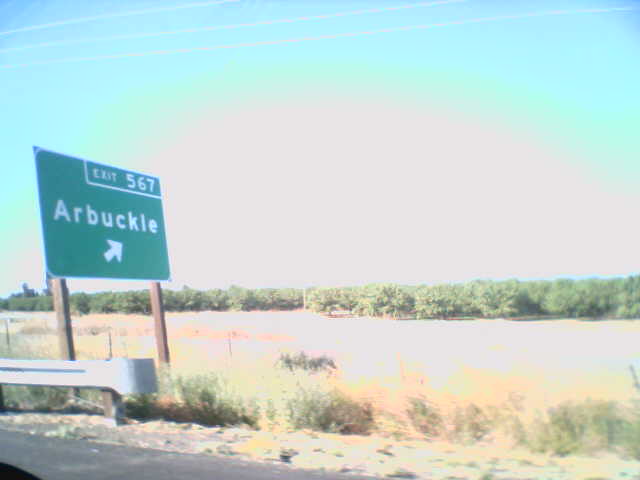A photograph of a highway scene captured from the passenger side window of a car. The bottom left corner of the image reveals a small portion of the car's interior and a segment of the guide rail running alongside the road. Dominating the center of the image is a green highway sign with white text that reads "Arbuckle" and an arrow pointing to the right. Above this, the sign indicates "Exit 567". The background displays a stretch of grassy area extending beyond the sign, contributing to the roadside setting. The overall composition of the photo directs attention to the highway sign, which is angled towards the right side of the frame.